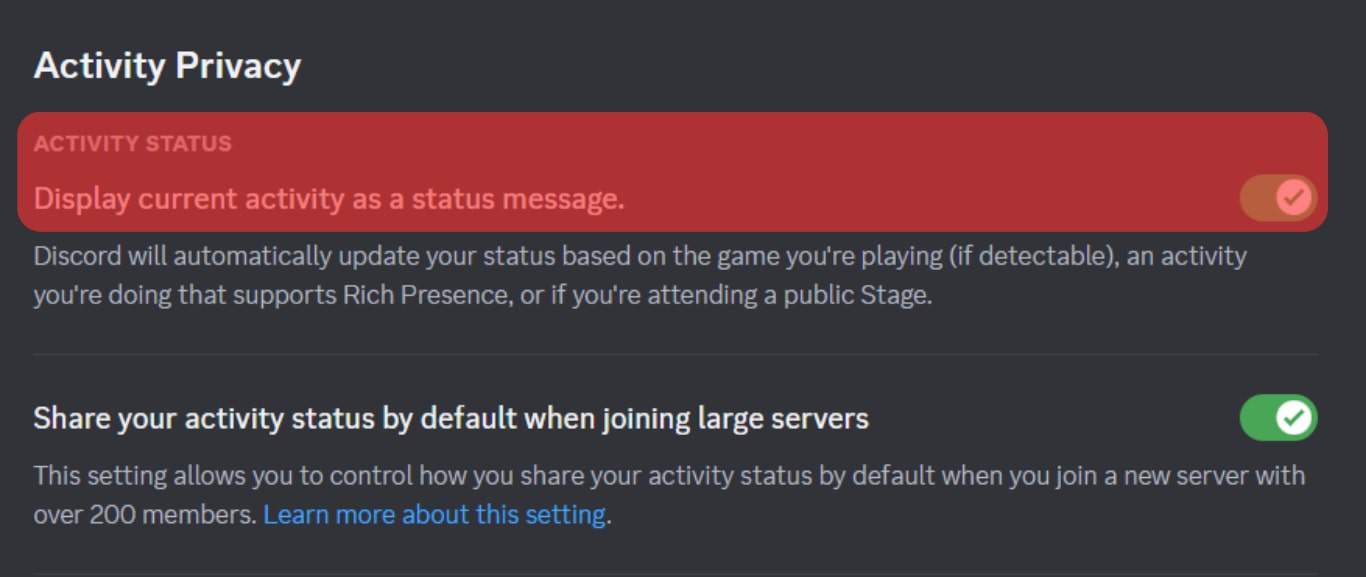The image features a pop-up notification titled "Activity Privacy," with a predominantly dark slate gray background accented by white text. The section for "Activity Status" is prominently highlighted in red, including the toggle switch, which is turned on. The description beneath explains that when enabled, Discord will automatically update the user's status based on detectable activities such as games, activities supporting rich presence, or attendance at public stages.

Below this, a divider separates the content, leading to another setting regarding the sharing of activity status by default when joining large servers. This subsection advises that with this setting turned on, users can control whether their activity statuses are shared upon joining servers with over 200 members. A blue hyperlink labeled "Learn more about this setting" is also present, likely offering additional information. This setting is currently enabled, as indicated by a green toggle switch with a checkmark.

The color scheme for the text includes shades of white, gray, blue, and red, with the red specifically highlighting the "Activity Status" section, providing a clear visual distinction. The overall design does not explicitly indicate the platform (website or mobile), but the layout and visual cues suggest a user interface typical of Discord.